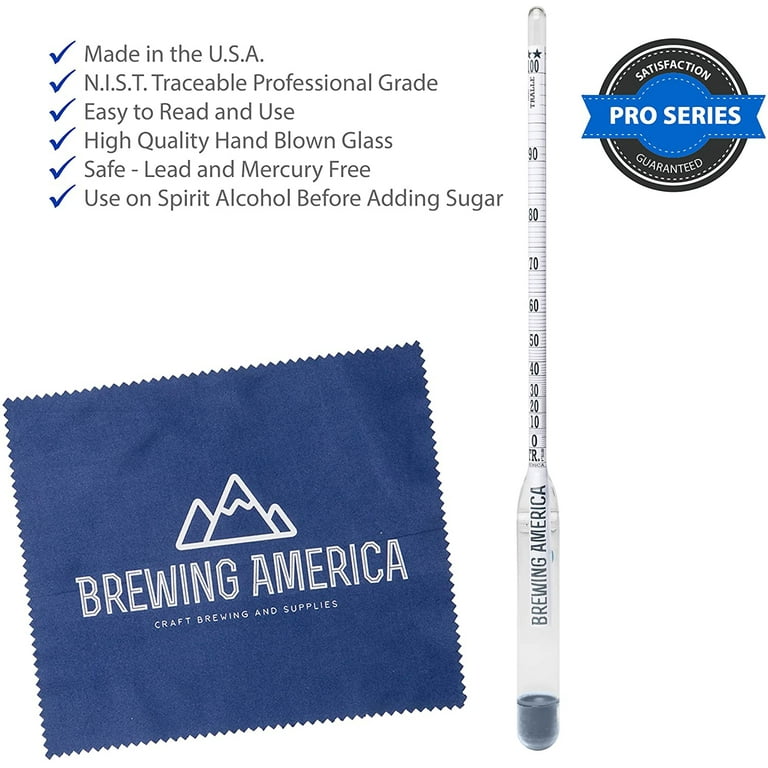This promotional image for Brewing America Craft Brewing and Supplies features a dark blue, square piece of fabric with serrated edges, measuring approximately two inches by two inches. Embroidered in the center are white line drawings of mountains, with the words "Brewing America Craft Brewing and Supplies" stitched below in block letters. A large, clear glass alcohol thermometer, labeled vertically with “Brewing America,” stands prominently in the middle. This high-quality hand-blown thermometer is marked with various measurement areas, with the top number reading 100 and surrounded by stars. A black circular logo with a blue ribbon in the center, stating “Satisfaction Pro Series Guaranteed,” is located in the upper right corner. On the left side of the image is a check-off list highlighting key features: "Made in the USA, NIST Traceable Professional Grade, Easy to read and use, High quality hand-blown glass, Safe, lead and mercury free. Use on spirit alcohol before adding sugar.”